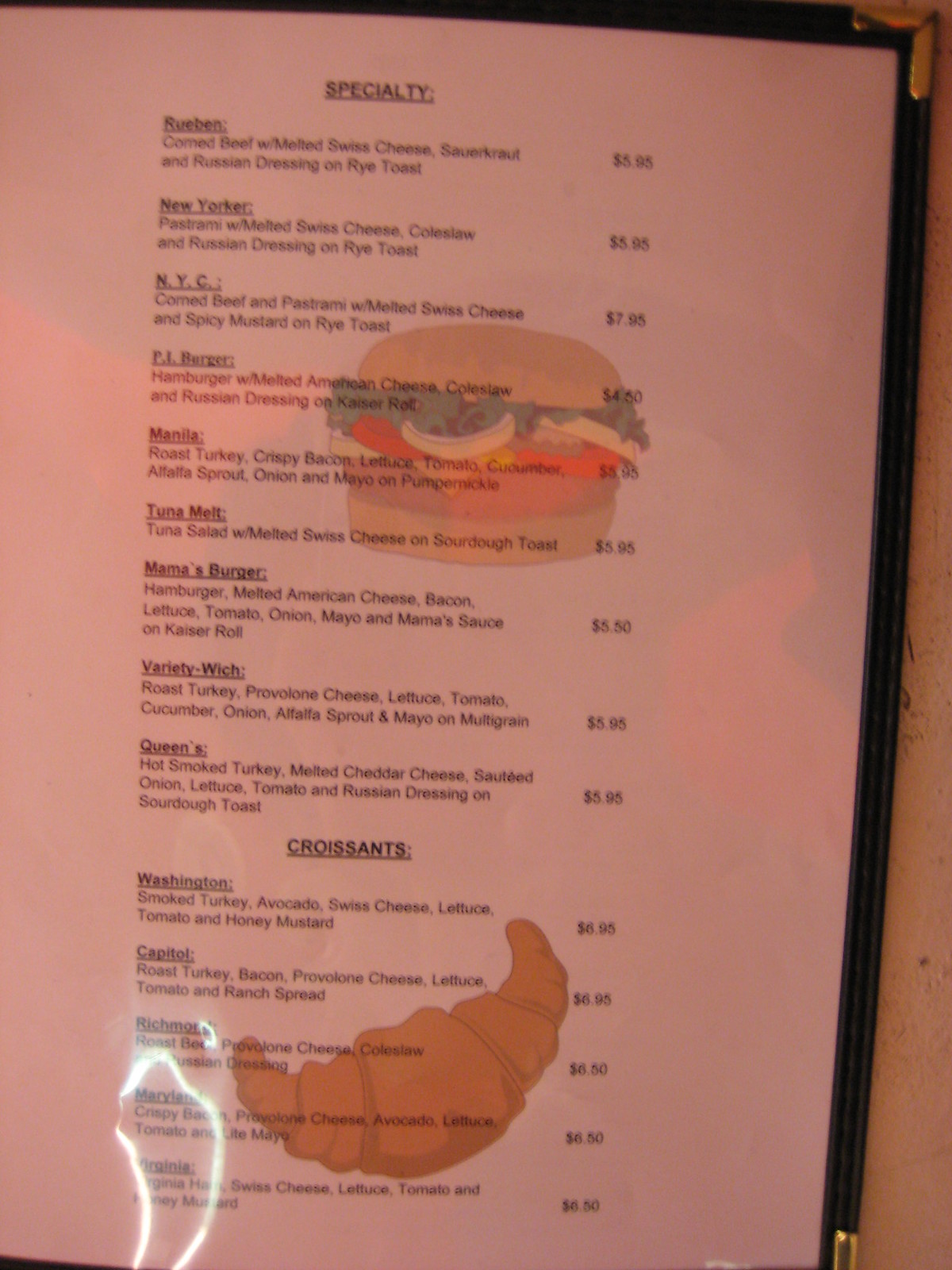The image displays a neatly designed menu page set against a light brown table. The menu has a distinguished border that resembles black leather, complete with gold metal tips at each corner, suggesting the backside could also be leather. Positioned centrally on the white page are two clipart images: a hamburger near the center and a croissant towards the bottom.

At the top of the page, the word "Specialty" is elegantly written in small black letters and underlined. Below this heading, various sandwiches are listed along with their ingredients and prices. The menu includes options such as "Reuben," "New Yorker," "NYC," "PJ Burgers," "Manila," "Tuna Melt," "Mama's Burgers," "Variety Wish," and "Queens," each detailed with their respective ingredients listed underneath and prices aligned to the right.

Further down, another section is dedicated to croissants, marked by the bold, underlined heading "Croissants." This section outlines several varieties: "Washington," "Capital," "Richmond," "Maryland," and "Virginia," with each croissant accompanied by a list of ingredients underneath and the price to the right.

The meticulous design and detailed descriptions on this elegant menu page suggest a sophisticated dining experience.